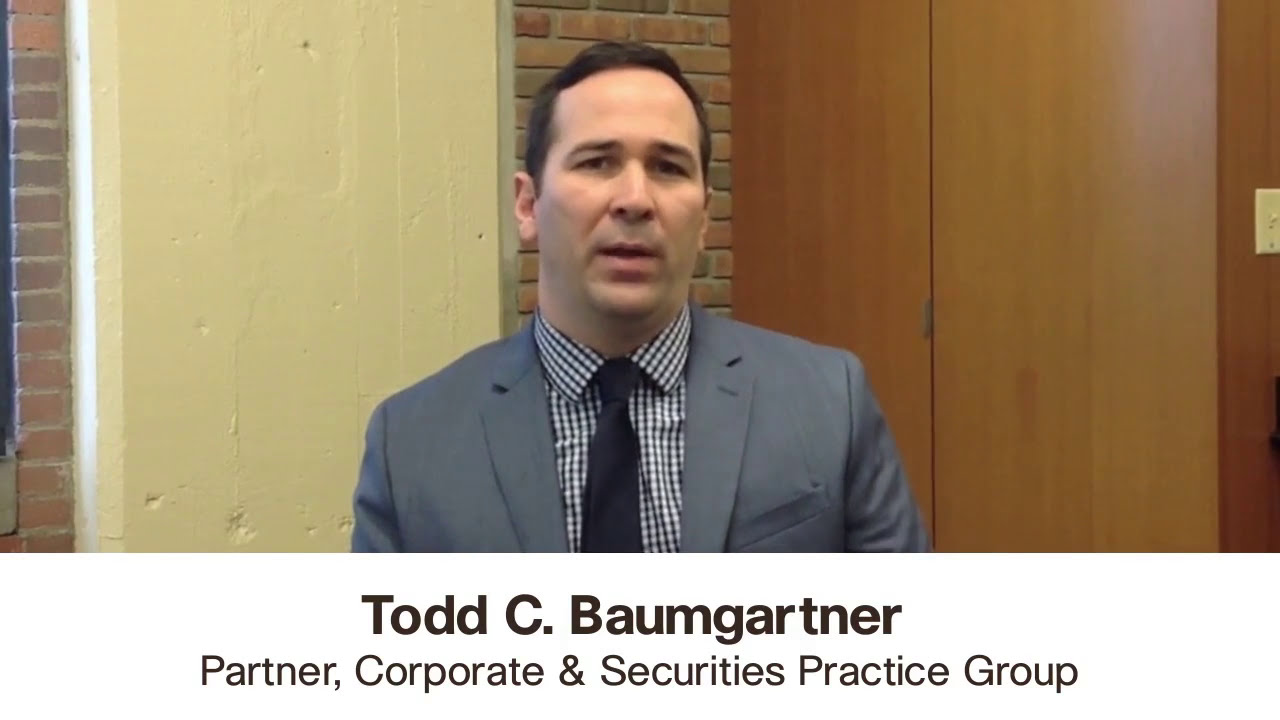The image features a white gentleman with short dark hair, dressed in a gray suit jacket, a checkered shirt, and a solid black tie. He is pictured from just below his chest to the top of his head, and he appears to be speaking, with his mouth partially open as if mid-sentence. He stands in front of a setting that includes a brick wall, a large door, and a light switch on the wooden wall to the right. Below the photo, in black lettering, the text reads: "Todd C. Baumgartner" and beneath it, "Partner, Corporate and Securities Practice Group." The text is prominently displayed, identifying him and his professional role.